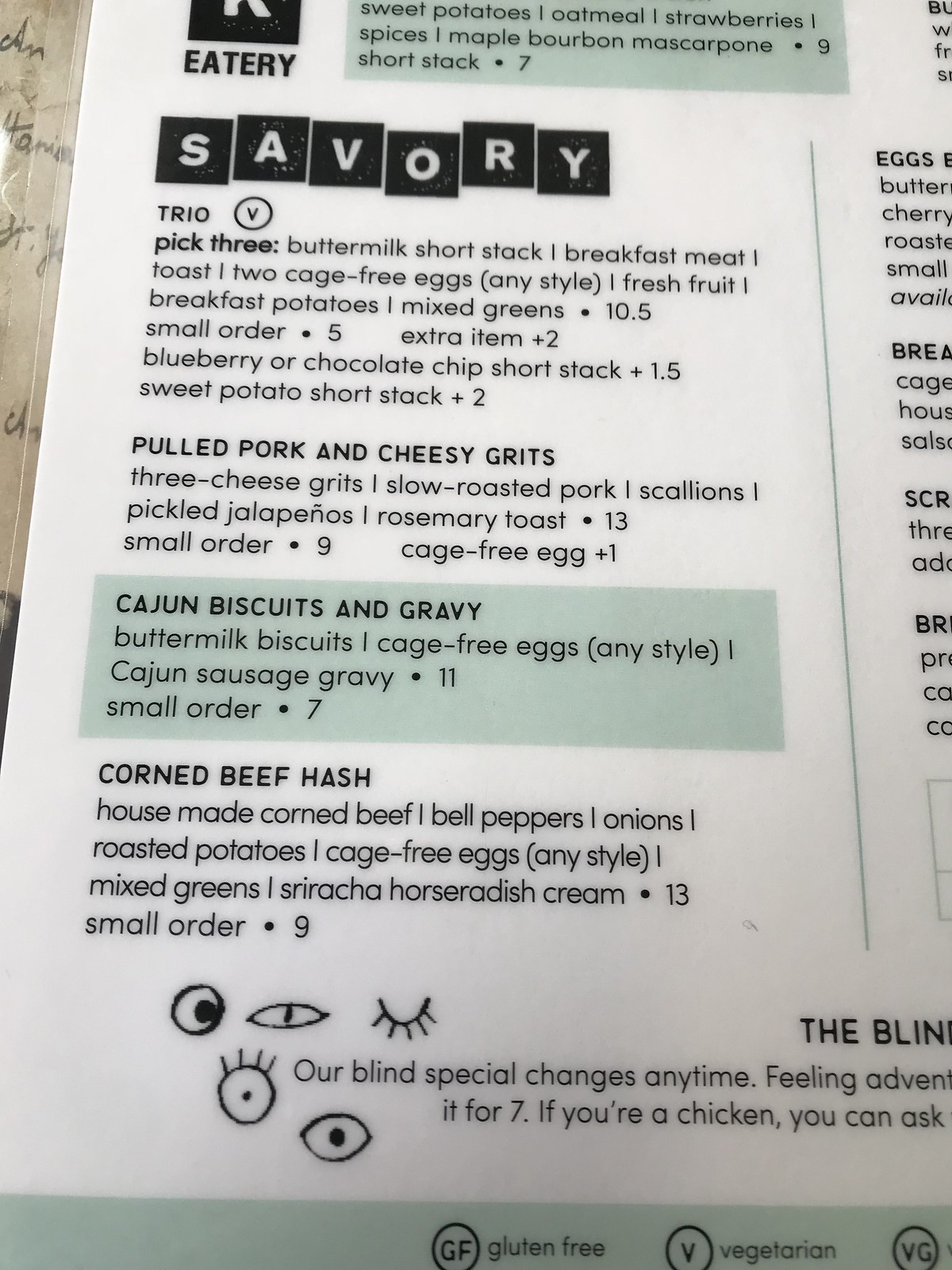This image captures a section of a white menu with black text and some grayish-green highlights. The visible portion shows the left side of the menu, which is cut off at the top and extends almost to the bottom of the page.

At the top left corner, the menu features the word "Eatery." Below this, within a partially visible grayish-green box, the beginning is cut off, but you can read a list of ingredients: "Sweet potatoes, oatmeal, strawberries, spices, maple bourbon, mascarpone."

Following this, the word "SAVORY" is prominently displayed, each letter encapsulated in a white font on black squares. The squares are vertically offset from each other and separated by thin white lines.

Underneath this section, there are several menu items. The first item listed is "Trio," which invites you to pick three choices. Next is "Pulled Pork and Cheesy Grits." Both these items are presented in black text on the white background. 

A highlighted gray-green section then names the dish "Cajun Biscuits and Gravy." Below that, in black text on white again, is "Corned Beef Hash." Each dish name is accompanied by a brief description of the ingredients or preparation method.

At the bottom of the visible section, there's partially obscured text mentioning something about a "blind special" that can change frequently, but the message cuts off before it can be fully read.